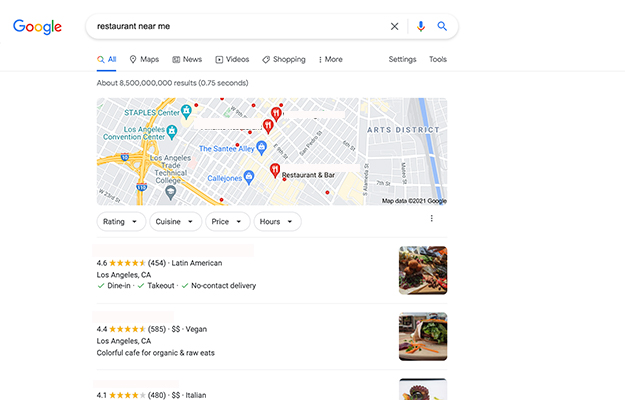**Detailed Caption: Screenshot of Google Search Results for "Restaurant Near Me"**

This image is a detailed screenshot of Google search results for the query "restaurant near me". The background is predominantly white. 

**Top Section:**
- At the top left, the Google logo is prominently displayed in its signature colors.
- Adjacent to the logo is the search bar with slightly rounded corners and a subtle shadow. It contains the search query "restaurant near me" in all lowercase black letters.
- On the far right of the search bar are three icons: an 'X' to clear the search field, a microphone for voice input, and a blue magnifying glass for initiating the search.

**Navigation Tabs:**
- Directly below the search bar is a horizontal menu of tabs starting from the left:
  - "All" (selected, in blue with a blue underline and a search icon).
  - "Maps" (with a location pin icon).
  - "News" (with a newspaper icon).
  - "Videos" (with a video camera icon).
  - "Shopping" (with a shopping tag icon).
  - A three-dot menu symbol followed by "More", and finally "Settings" and "Tools".

**Search Information:**
- Beneath these tabs, there is a thin gray line followed by search result metadata stating "About 8,500,000,000 results (0.75 seconds)".

**Map and Filters:**
- The map below this metadata shows a section of Los Angeles with notable landmarks such as the Staples Center, Los Angeles Convention Center, Los Angeles Trade Technical College, Callejones (Santee Alley), a Restaurant Bar, and the Arts District. The map is marked with three red location pins.
- Below the map, there are four filter ovals: 
  - "Rating", "Cuisine", "Price", and "Hours".

**Listed Search Results:**
- A thin gray line demarcates the section with actual search results. The results visible in the image are:
  1. **First Result:** 
     - Displays a rating of 4.6 stars, with 454 reviews in parentheses.
     - "Latin American" cuisine in Los Angeles, California.
     - Features checkmarks indicating "Dine-in", "Takeout", and "No-contact delivery".
     - A thumbnail image of the restaurant is shown on the far right.
  2. **Second Result:**
     - A vegan restaurant with a 4.4 star rating.
     - Includes similar attributes and a thumbnail image.
  3. **Third Result (Partially Visible):**
     - Has a 4.1 star rating and a partially visible thumbnail image.

This screenshot provides a thorough overview of a typical search result page on Google for restaurants in a specified area, emphasizing the map, navigation tabs, and user ratings.